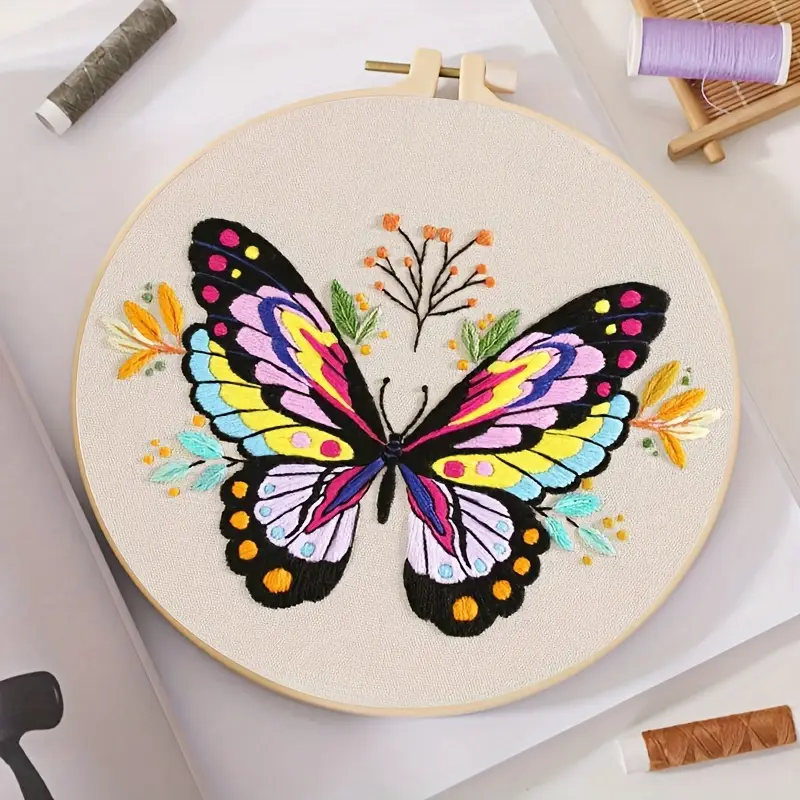This image showcases an intricately detailed and colorful cross-stitch embroidery of a butterfly mounted on a circular ring. The butterfly, meticulously crafted with threads of various hues, features black wings adorned with layers of vibrant pink, yellow, light and dark purple closer to the center, transitioning into a darker pink near the middle. The wings are beautifully accentuated with multicolored dots - darker pink and yellow on the top wings, with similar yellow against the darker shades on the bottom wings. Surrounding this lifelike butterfly are leaf-shaped patterns embroidered in a harmonious mix of yellow, blue, and green threads, filling in the negative space and adding to the overall design's aesthetic appeal.

The embroidery piece is staged on a pristine white surface, likely a table or a couch, making for a picture-perfect setting that's highly suitable for platforms like Instagram or Pinterest. Few spools of thread are thoughtfully placed around the piece, enhancing the visual appeal of the scene. The finished embroidery remains within its hoop, maintaining a tidy and traditional presentation. This project, with its striking and detailed depiction of the butterfly and the accompanying leaves, demonstrates considerable skill and artistry, making it a truly captivating piece.